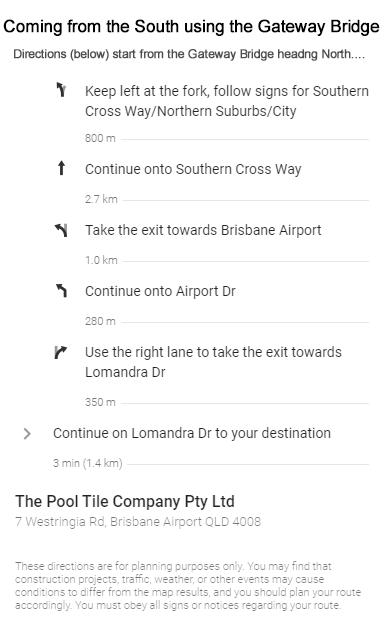**Driving Directions to The Poole Tile Company PTY LTD**

**Starting Point:** Gateway Bridge (Heading North)

1. **Keep Left at the Fork:** Follow signs for Southern Crossway, Northern Suburbs, and City (800 meters). 

   ![Arrow pointing up and slightly to the left]

2. **Continue on Southern Crossway:** Travel straight for 2.7 kilometers.

   ![Arrow pointing straight up]

3. **Take the Exit:** Towards Brisbane Airport (1.0 kilometer). 

   ![Arrow pointing left, up and to the left]

4. **Continue on Airport Drive:** For 280 meters after the exit.

   ![Arrow pointing upwards and to the left]

5. **Use Right Lane:** Take the exit towards Lomandra Drive (350 meters). 

   ![Arrow pointing up and to the right]

6. **Continue on Lomandra Drive:** Travel for 1.4 kilometers to your destination.

   ![Arrow pointing right]

**Destination:** The Poole Tile Company PTY LTD, 7 West Stringia Road, Brisbane Airport, QLD, 4008.

**Note:** These directions are for planning purposes only. Construction projects, traffic, weather, or other events may affect actual conditions. Always obey all road signs and notices. Plan your route accordingly.